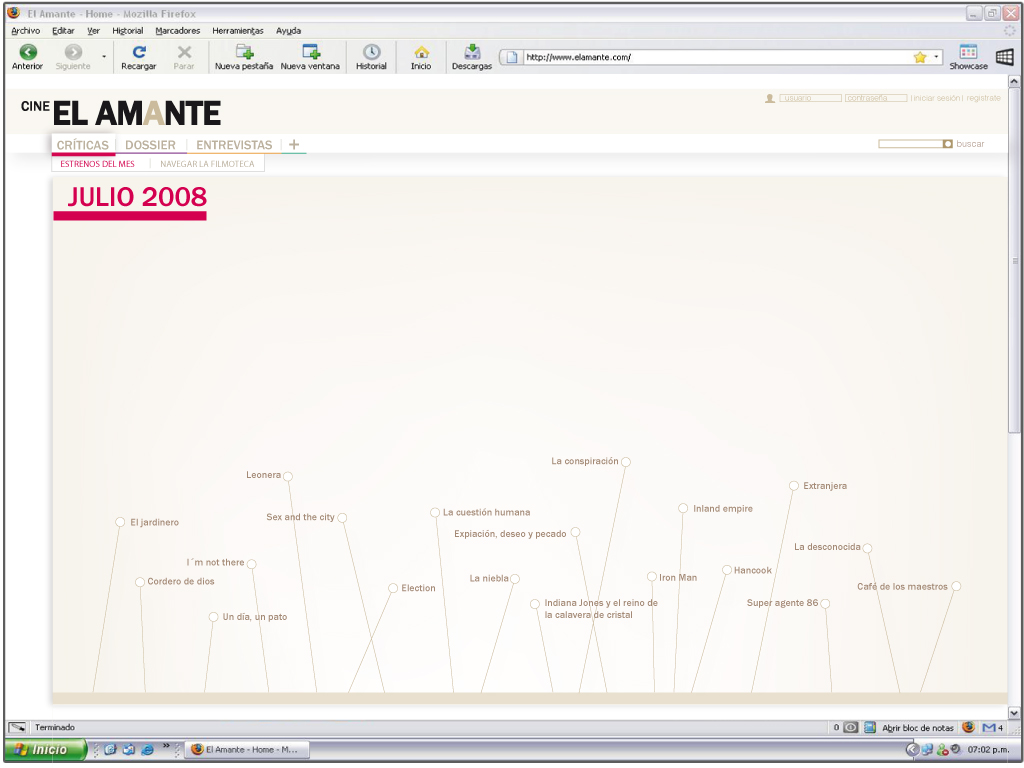This image is a screenshot from an older version of Windows, likely Windows XP or Windows Vista, running on an older version of Firefox, dating back to around 2008. The screenshot showcases a web page from elamante.com, a Spanish-language website, as indicated by text such as "Julio 2008" and the "Inicio" button on the taskbar. The webpage header features “Cine El Amante” in bold black letters beneath which there’s a pink banner displaying "Julio 2008". The background is grey with graphical elements consisting of lines ascending from the bottom, culminating in white circles adjacent to various phrases and titles. These titles include "I'm Not There", "Sex and the City", "Iron Man", "Inland Empire", "Super Adventure 88", "Indiana Jones", "Hancock", and "Election". These labels, possibly denoting events or film releases on particular dates, are placed at different points along the graphical lines. The overall design suggests that this webpage might serve as a calendar or schedule, listing significant happenings or movie premieres for that period, with most text presented in Spanish.